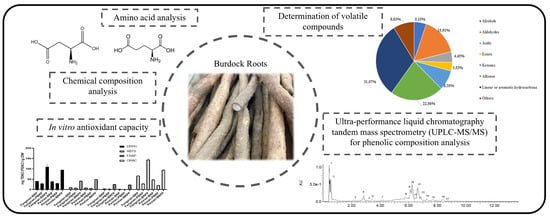The image is a horizontally aligned rectangular diagram with a black border and rounded corners, set against a white background. At the top left, it features the title "Amino Acid Analysis" within a dashed line, accompanied by illustrations of two different molecules. Directly below, another dashed line contains the title "Chemical Composition Analysis." Following this, the description "In Vitro Antioxidant Capacity" appears with a corresponding bar chart at the bottom. Central to the diagram is a circular dashed line labeled "Burdock Roots," showing several long, brown roots, one of which is cut open to reveal its interior. To the right of this circular section, the title "Determination of Volatile Compounds" is displayed within another dashed line, next to a colorful pie chart. Below this, yet another dashed section presents the title "Ultra-Performance Liquid Chromatography, Tandem Mass Spectrometry for Phenolic Composition Analysis," accompanied by a scatter chart underneath.